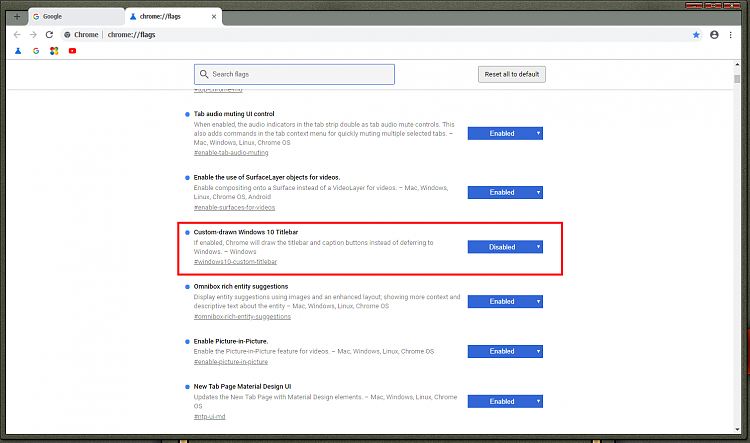This image depicts the search area page of a website, specifically a configuration or settings page for Google Chrome flags. At the top of the page, there are two folder icons: the left one labeled "Google" which is closed, and the right one, which is open, potentially labeled "Chrome" and possibly "tags". 

The address bar at the top reads "chrome://flags", indicating the user is on the experimental features page of Google Chrome. To the left of the URL, navigational arrows are present—one pointing left and another pointing right—followed by a refresh icon. To the right of the address bar, a blue star icon, an empty profile avatar, and a three-dot menu are visible.

Below the address bar, there are four Google-related icons and a search box containing an icon. Alongside the search box, a "Reset all to default" button is displayed. Beneath this line, a series of bulleted items are listed, with the third item highlighted in relation to Windows 10. This item has a red box drawn around it, indicating it is selected, and a drop-down menu next to it is set to "Disabled".

This detailed interface suggests the user is exploring different experimental features or flags within the Chrome browser settings, possibly for testing or configuring browser behavior.